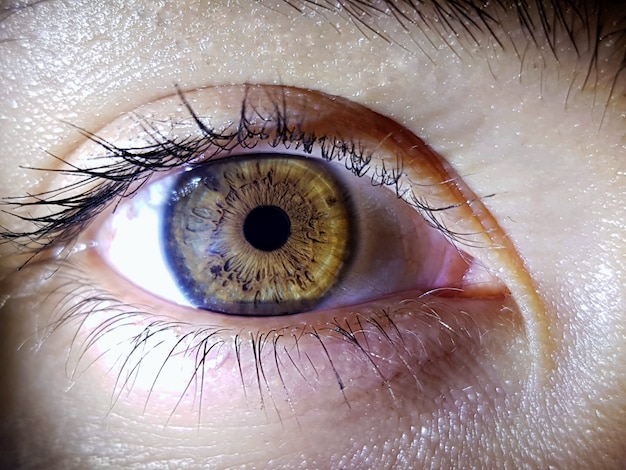This professional, close-up photograph captures an eye with meticulous detail. The eye, slightly off-center towards the left, is open to a regular amount, revealing intricate features. The iris displays a greenish-hazel hue with flecks of yellowish brown and dark speckles, creating a dramatic and arrayed effect. Surrounding the iris, the dark brown outline contrasts with the dark black pupil at its center. The sclera, or the whites of the eye, may have a slight brownish smudge, though it could be a shadow or light trick. The eye is framed by dark, distinct top and bottom lashes, and part of the eyebrow emerging from the top. The fair skin around the eye, possibly lightened by a glare, showcases the porous texture and folds of the eyelid. The precise light and shadow create a dramatic visual emphasis on the detailed and expressive eye.